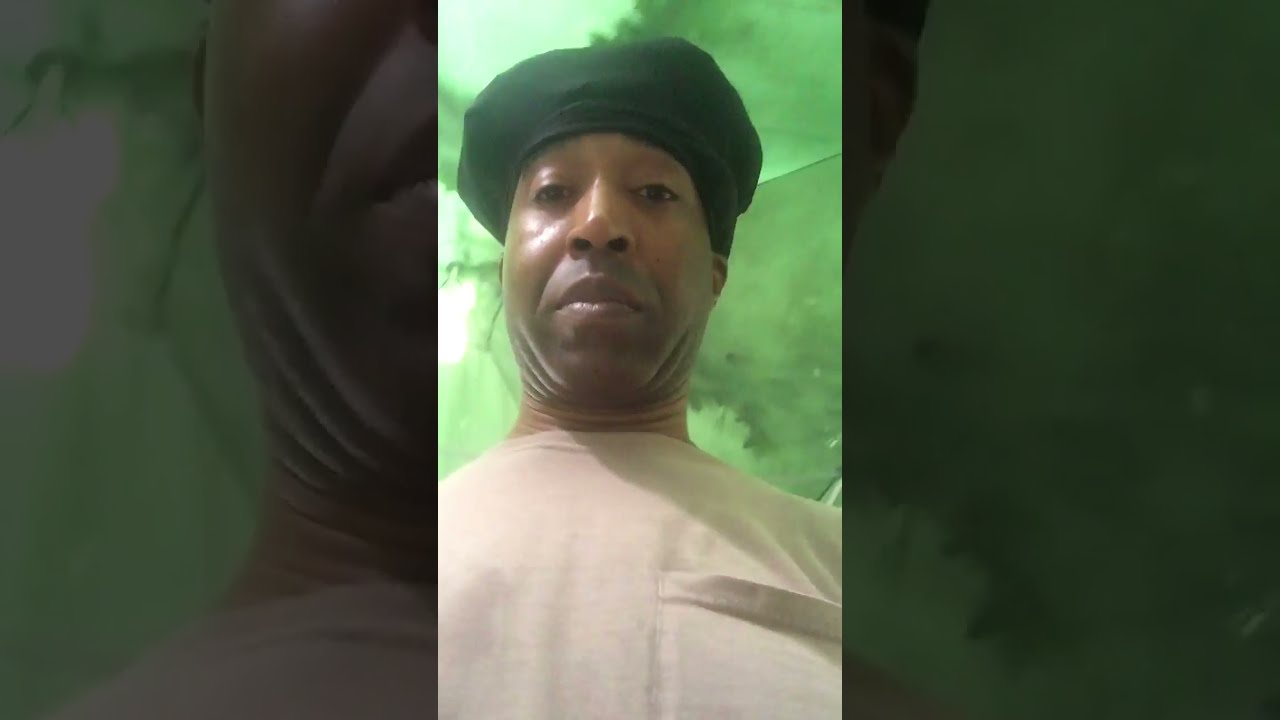The image is divided into three segments with distinct filters. In the center is a selfie of an African-American man, gazing at the camera with a neutral expression. He is wearing a beige t-shirt with a pocket on the lapel and a black head wrap. Behind him is a pale green backdrop that appears hazy with hints of leaves or smog. The segments on the right and left side of the image are filtered and darkened. The left segment provides a close-up of the man's face, focusing on his nose and lips, highlighting his wide nose and prominent upper lip. The right segment, while blurry and harder to distinguish, also seems to feature a filtered portion of the man or the backdrop, maintaining the overall darkened aesthetic.